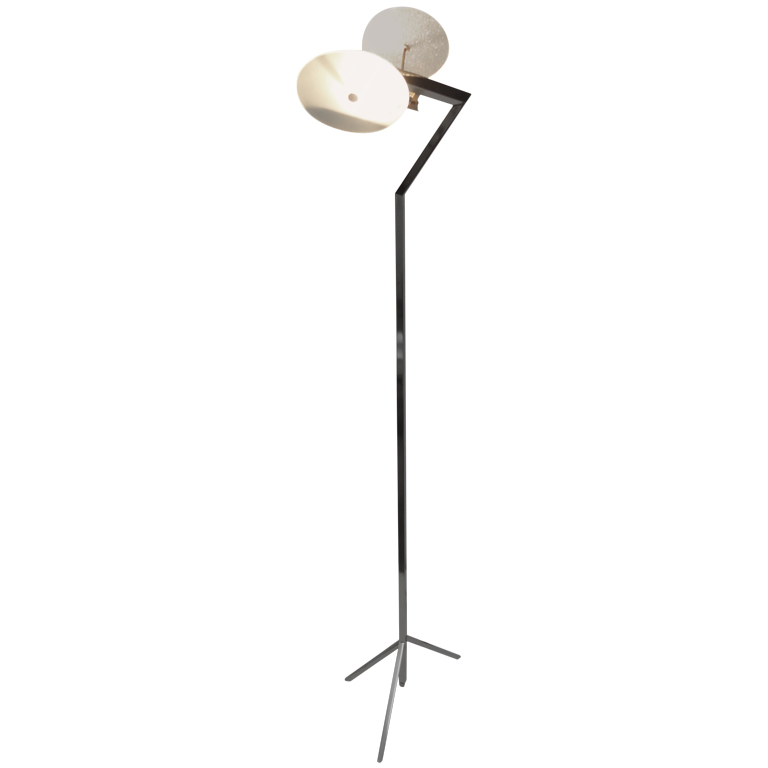This photograph features a tall metal stand with a varying coloration from a lighter grey base transitioning to a darker top. The stand is supported by multiple legs, likely three or four, to ensure stability. At the top of this stand, there is a horizontal bar that holds two circular, white discs that resemble buttons or possibly light fixtures, although their exact function is unclear. These discs are connected to the stand with gold or copper-colored rods and are arranged to face each other. The structure has a slight hook-like bend at the top, adding to its intricate appearance. The overall height of the stand is estimated to be around four feet, making it a prominent and somewhat mysterious instrument, possibly resembling scientific equipment.